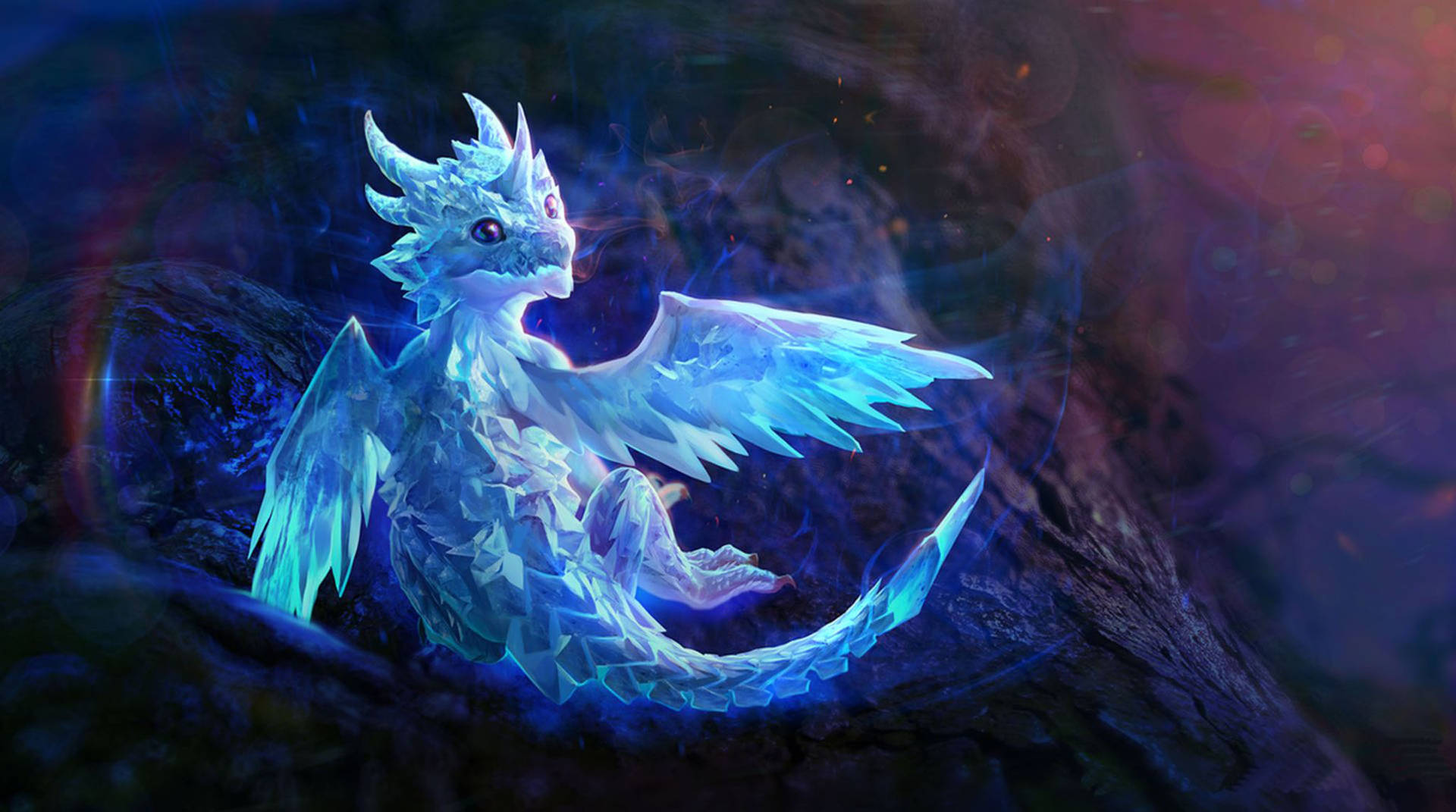This vibrant, highly detailed digital painting showcases a baby ice dragon, intricately designed with craggy, light blue scales and feathery icy wings. The dragon displays an inquisitive demeanor, lying on its back with its belly exposed and tail curling up, as it gazes over its shoulder. Its head is adorned with several icy horns, including a rhinoceros-like horn on its nose. The background is a colorful gradient tapestry, transitioning from red with hints of gold and lighter reds in the upper right corner, down to dark blue, dark gray, and black at the bottom. Colorful patches of green and blue intersperse the lower left side, adding to the scene's richness. The dragon rests on a realistic-looking log, further enhanced by a stylized digital lens flare and halo of light, creating a harmonious fusion of fantasy and realism. The overall tones beautifully blend light blue hues for the ice dragon with darker blue and purple-red shades for the background.